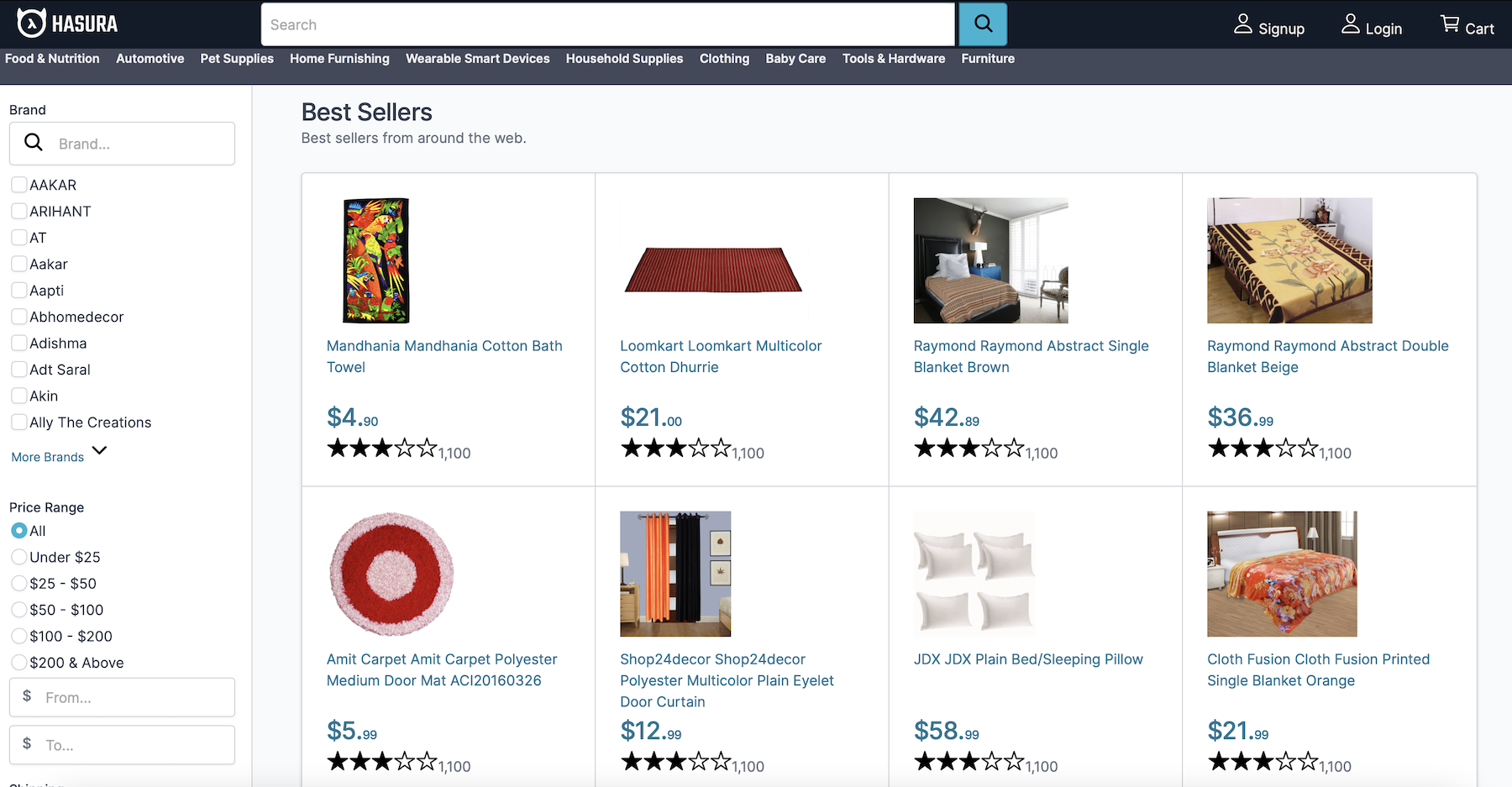The image is a screenshot of an e-commerce website with a design reminiscent of Amazon's layout. The upper portion of the site features a navy blue border. On the left side of this border, the brand name 'Hasura' is displayed in white text. Adjacent to the brand name is a white search bar, accompanied by a blue icon with a magnifying glass symbol. On the far right, the options to "Sign Up," "Log In," and access the "Cart" are available.

Below the main border, a gray navigation bar lists various product categories: Food and Nutrition, Automotive, Pet Supplies, Home Furnishing, Wearable Smart Devices, Household Supplies, Clothing, Baby Care, Tools and Hardware, and Furniture.

The main section of the webpage, set against a white background, highlights the "Best Sellers" and "Best Sellers from Around the Web." Various products, both named and imaged, are displayed:

1. Madhania Cotton Bathtowel - $4.90
2. Loom Cart Multicolor Cotton Durry - $21.00
3. Raymond Abstract Single Blanket in Brown - $42.89
4. Raymond Abstract Double Blanket in Beige - $36.99
5. Amit Carpet Medium Door Mat (AC120160326) - $5.99
6. Shop 24 Div Core Polyester Multicolor Plain Eyelet Door Curtain - $12.99
7. JVX Plain Bed Sleeping Pillow - $58.99
8. Cloth Fusion Printed Single Blanket in Orange - $21.99

The website likely offers a broad range of products with detailed listings and images to guide potential buyers.